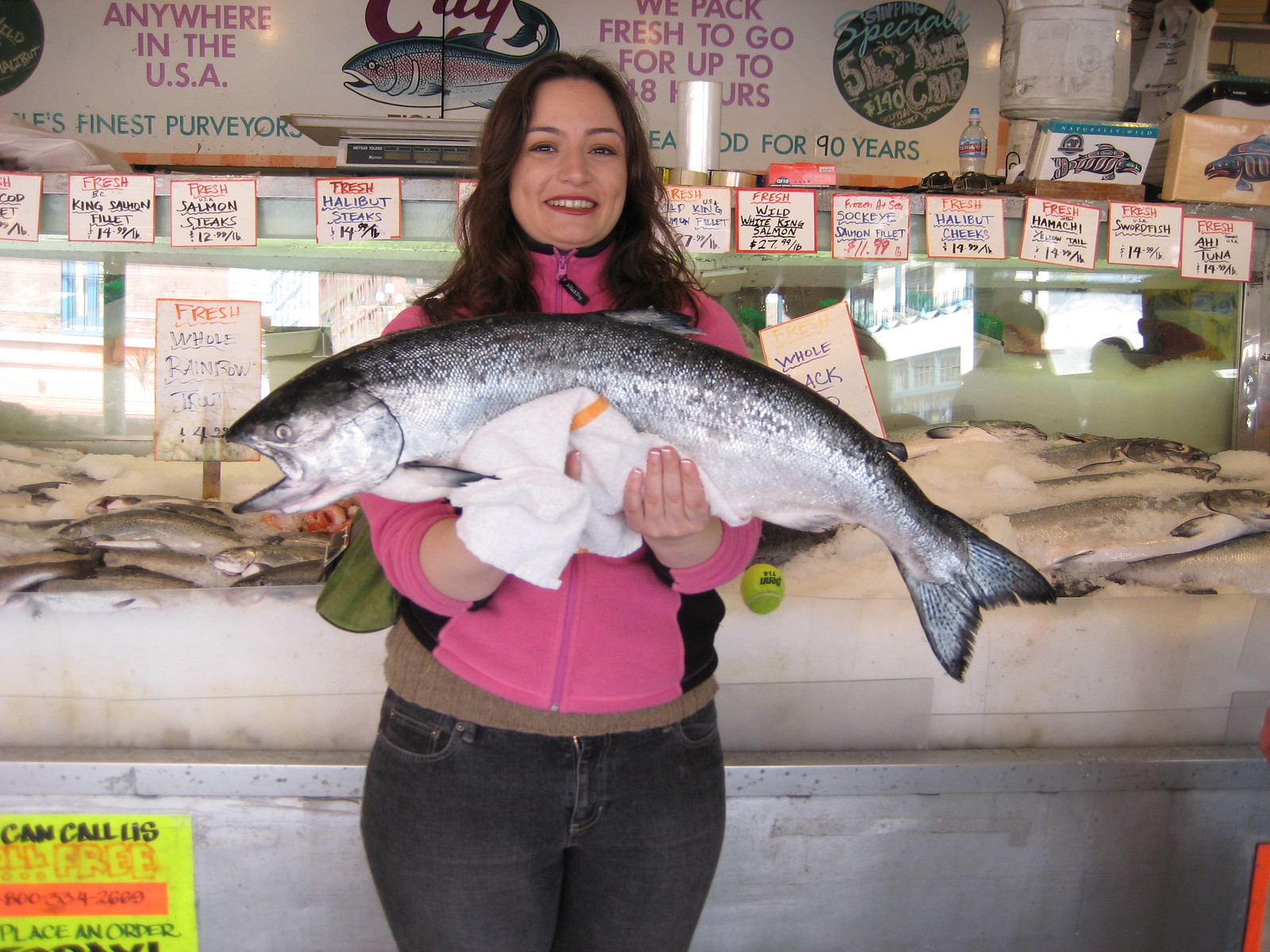In this detailed photograph, a smiling woman with long brown hair and dimples is energetically holding a massive, shiny silver fish with its mouth open, pointed to the left. She is dressed in a layered outfit consisting of a pink sweater over a brown sweater, coupled with blue jeans, and possibly has a green backpack or purse behind her. Using a towel to grip the fish, she holds it with her palms facing up. The setting is a bustling fish market, evidenced by the background showcasing a shelf filled with ice and various whole fish on display. Above the shelf, numerous placards detail the types and prices of the fish, with descriptions written in black, blue, and red marker. Prominent signs above the placards include messages such as "Anywhere in the USA, finest purveyors" and "We pack fresh to go for up to 48 hours," underscoring the market’s commitment to quality and freshness. The atmosphere is lively and professional, capturing the essence of a market known for its premium seafood offerings.